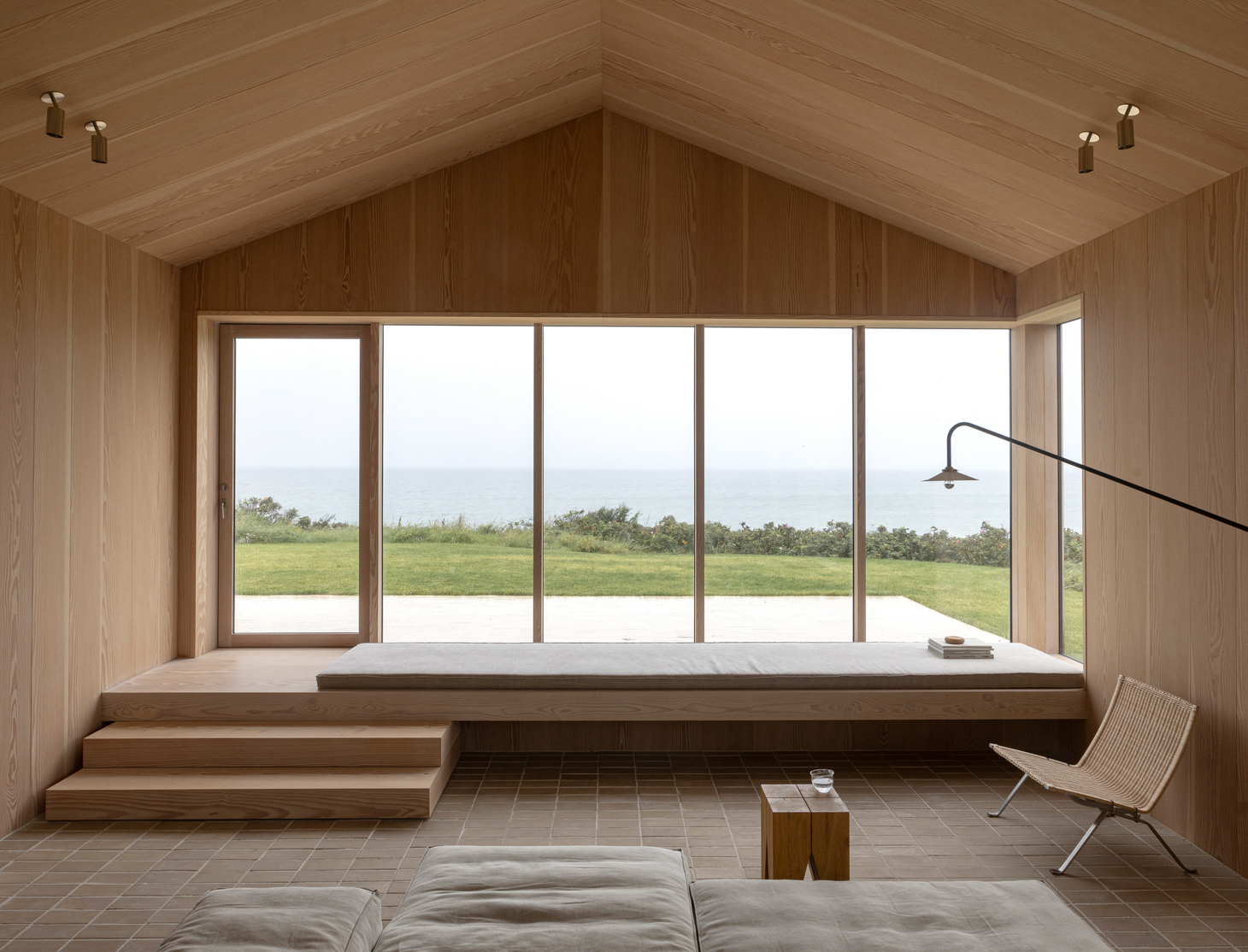This photograph captures a spacious room with high, wooden-paneled walls and ceiling, complemented by a beige tile or brick floor. The far end of the room features a striking wall of windows, one of which is a door, that opens onto a large cement patio. Beyond the patio, a lush green lawn, scrubby bushes, and a body of water—possibly an ocean or a large lake—are visible in the distance under a cloudy sky. Inside, the room is furnished with several large and fluffy mats on the floor, a small wicker bench, and a wooden table holding a glass of water. There are three steps leading up to a raised wooden area with a large gray pad on it, which holds a tray. The serene and airy ambiance of the room is emphasized by the natural light streaming in through the expansive windows.